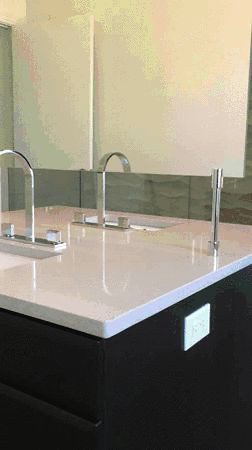The image captures a modern bathroom sink setup within a rectangular frame. The countertop, made of pristine white marble, exudes elegance and is seamlessly integrated with a sleek, silver metal sink faucet and matching handles, designed with a contemporary, hook-like shape. Below the countertop, there are black drawers that create a striking contrast, continuing the sophisticated monotone palette with black-painted sides. 

On the side of the counter, a standard white electrical outlet is visible, adding a functional touch to the scene. The countertop also features a reflective mirror mounted on the wall, which provides a glimpse of additional white and gray wall panels and echoes the image of a door positioned on the left. To the right of the countertop, a metal bar, possibly a towel rack, is affixed, adding to the utility of the space. The upper corners of the wall appear to be white, while the mirror's reflection reveals gray wall panels beneath the white upper sections, contributing to the room's refined and harmonious design.